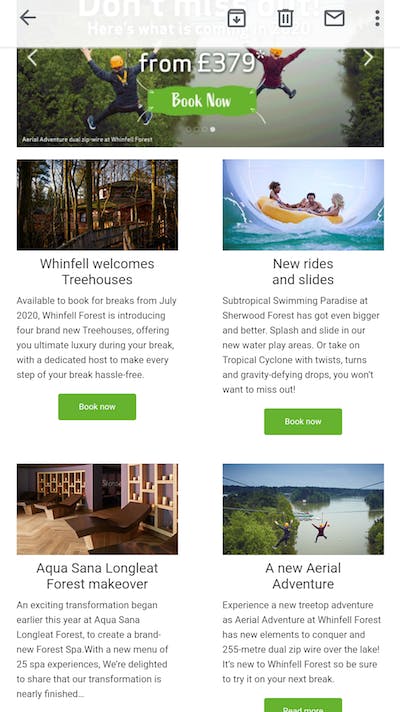Category: Websites

At the top of the webpage, there is a faded banner that reads "Don't miss out," positioned in the background. Below this banner, there are several icons: a back arrow, a download arrow, a trash can, an email icon, and a menu with three dots.

The main section features a vibrant image of two people mid-fall, bungee jumping above a body of water with lush greenery on either side. A promotional text overlay reads, "From £379. Book now."

Below this image, there's a caption discussing Winfell Forest's new offerings: "Winfell welcomes treehouses. Available to book for breaks from July 2020. Winfell Forest is introducing four brand new treehouses offering you the ultimate luxury during your break with a dedicated host who make every..." The text cuts off here, suggesting more information on these luxury offerings is available on the website.

Adjacent to the bungee jumping image, there's a dynamic photo of a group of people in a raft, emerging from a giant tube into water. The accompanying caption promotes new attractions: "New rides and slides. Subtropical Swimming Paradise at Sherwood Forest has got even bigger and better. Splash and slide in our new water play areas or take on the Tropical Cyclone with its twists and turns. There is also the Aquasana Longleaf Forest Makeover and a new aerial adventure."

This webpage showcases exciting adventure activities and luxurious accommodations, aimed at enticing visitors with thrilling experiences and unparalleled comfort.